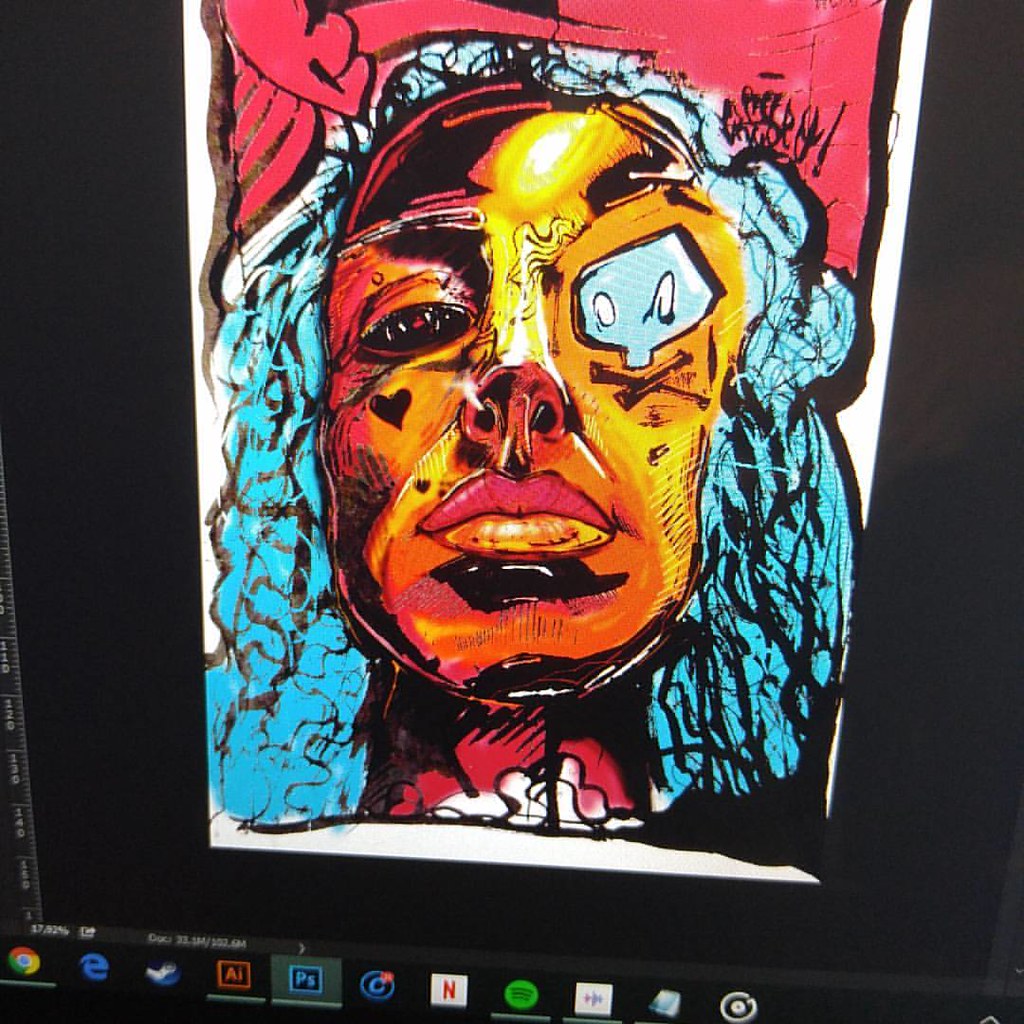Captured in this image is a screenshot of a computer desktop adorned with various application icons along the bottom. The visible icons include Google Chrome, Internet Explorer, Steam, an AI application, Adobe Photoshop (PS), a blue circle with a 'C' inside, Netflix, Spotify, and a few others that are not clearly identifiable. Dominating the screen is an evocative, artsy digital illustration featuring the face of a black woman. Her striking hair is rendered in neon blue, accentuated by a pink accessory, which resembles a towel but is likely something more artistic. The style of the illustration has a street art flair, reminiscent of the vibrant, expressive murals that grace urban environments, yet it is encapsulated within the boundaries of a computer screen.